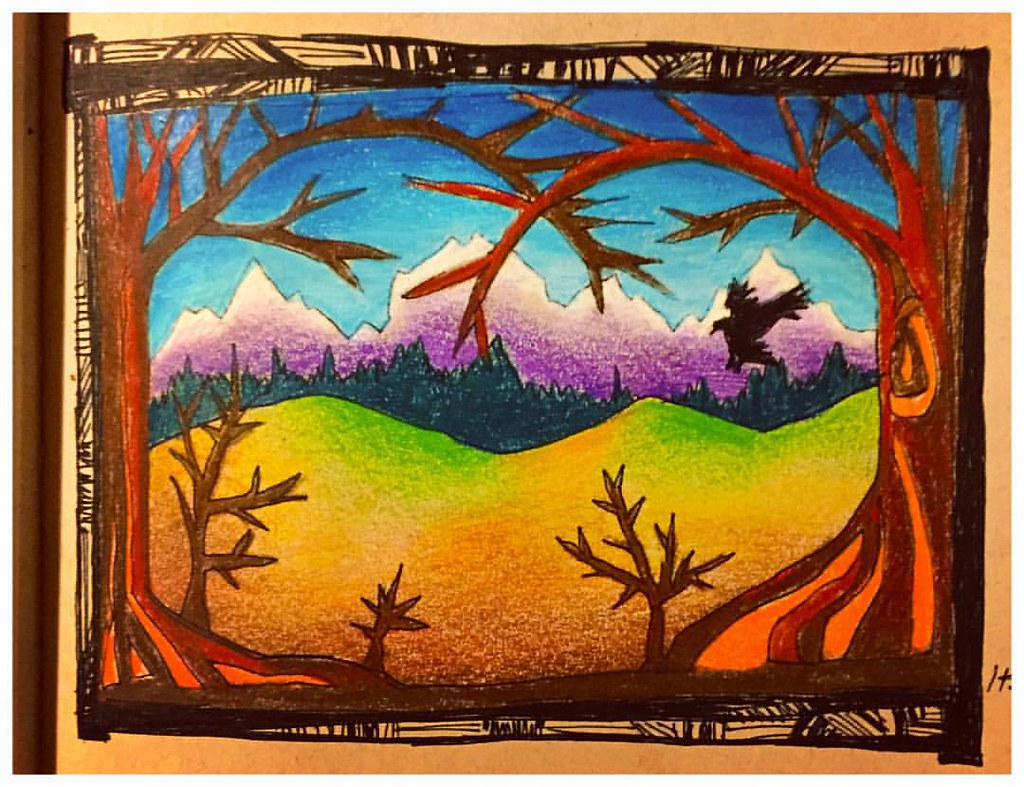This image features a detailed photograph of a drawing, depicting a picturesque landscape scene on white paper. Surrounding the drawing is a bold, black border adorned with geometric designs, adding a structured frame to the artwork. Within this frame, two trees, one on the left and the other on the right, with brown bark and gracefully arching branches, extend towards the center, creating a natural archway that frames the scene. 

In the foreground, a lush area of yellow and green grass stretches across the landscape, adding vibrancy to the scene. Beyond the grass, a distant outline of green trees creates a middle ground that separates the foreground from the majestic mountainous backdrop. The mountains, rendered in soft hues of purple and white, rise gracefully, adding depth and grandeur to the composition. Above the mountains, a serene blue sky completes the scene, lending a sense of tranquility and vastness to the overall image. This detailed and thoughtfully composed drawing brilliantly captures the serene beauty of a mountainous landscape.